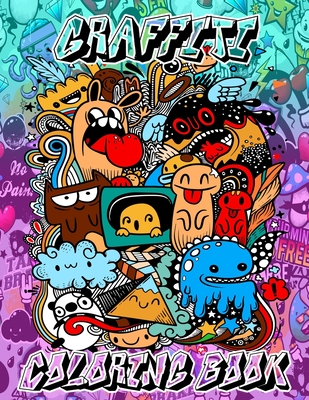This vibrant and captivating poster serves as the cover for a coloring book. Dominated by numerous colors, the top portion features "Graffiti" in a bold, graffiti-style font with turquoise and dark green accents. At the bottom, the words "Coloring Book" are similarly stylized with a purple-pink hue and dark purple accents, boasting a heavily 3D effect and shaded black edges.

In the center, a dense cluster of diverse and playful cartoon characters takes the spotlight. These characters include an exaggerated cartoonish dog, a cat, a cloud, and a quirky little figure inside a television set, among other silly and surreal creatures like a triangle with a smiley face. The characters are hand-drawn and exhibit a crazy, imaginative artwork style.

The background of the poster enhances its dynamic feel, with the top half predominantly featuring a cyan blue gradient and the bottom half showcasing a gradient purple backdrop. Additionally, more cartoon characters appear in the background, spaced out to create a sense of depth and chaos. The entire scene reflects a vibrant collage of hand-drawn and graffiti artworks, making it a visually stimulating feast for the eyes.